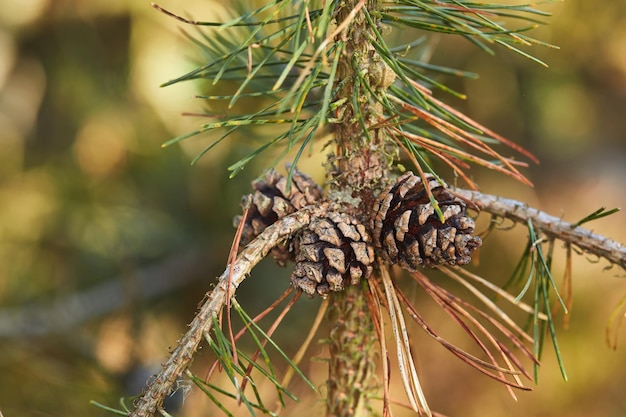This close-up photograph captures a pine tree branch in the woods, focusing intensely on three small pine cones that remain attached to the branch, suggesting they have not yet matured enough to fall off. Surrounding the pine cones, clusters of green pine needles dominate the scene, sprouting from two smaller offshoot branches. The pine cones exhibit a somewhat aged and faded appearance, with a mixture of light and dark green hues, as well as hints of light brown and yellow, indicating some needles may be drying or aging. The blurred background reveals a palette of greens, yellows, and blacks, indicative of a dense woodland setting, although it is indistinct and out of focus to accentuate the detailed foreground. The photograph, taken during daylight hours, deliberately obscures the background to highlight the pristine pine needles and cones, devoid of any people or text, thereby spotlighting the natural elements of the scene.